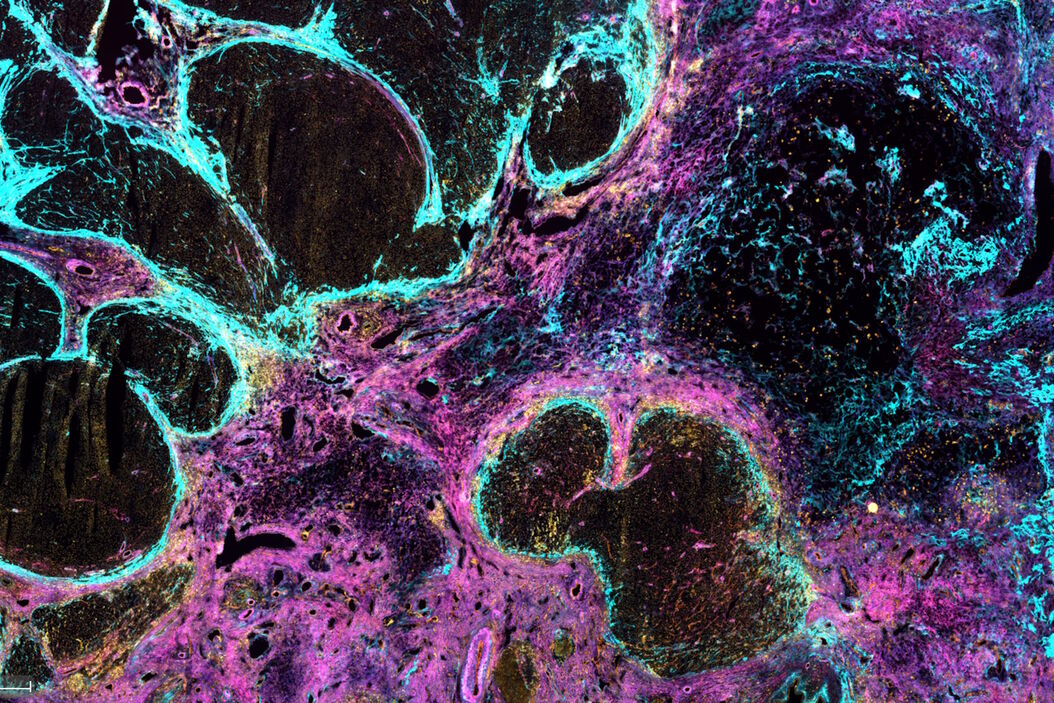The image features an abstract and vibrant piece of art that is both visually captivating and somewhat enigmatic. Dominated by swirling, asymmetrical shapes and circular objects, the composition is marked by a vivid combination of colors. The canvas is alive with splashes of pink, cyan, and coral, accented by occasional black patches, creating a contrast that pops against what appears to be a dark or black background. The painting exhibits a sense of organic randomness, with colors bleeding into one another, giving off an almost igneous or naturally occurring appearance. The intricate use of blue outlines around various shapes, coupled with expansive areas dominated by pink and coral hues, lends the artwork a neon, almost otherworldly glow. Despite its chaotic arrangement, the piece is visually cohesive and arresting, offering an intriguing blend of sickly yet bright colors that evoke a sense of natural phenomena, whether that be microbial, oceanic, or celestial.